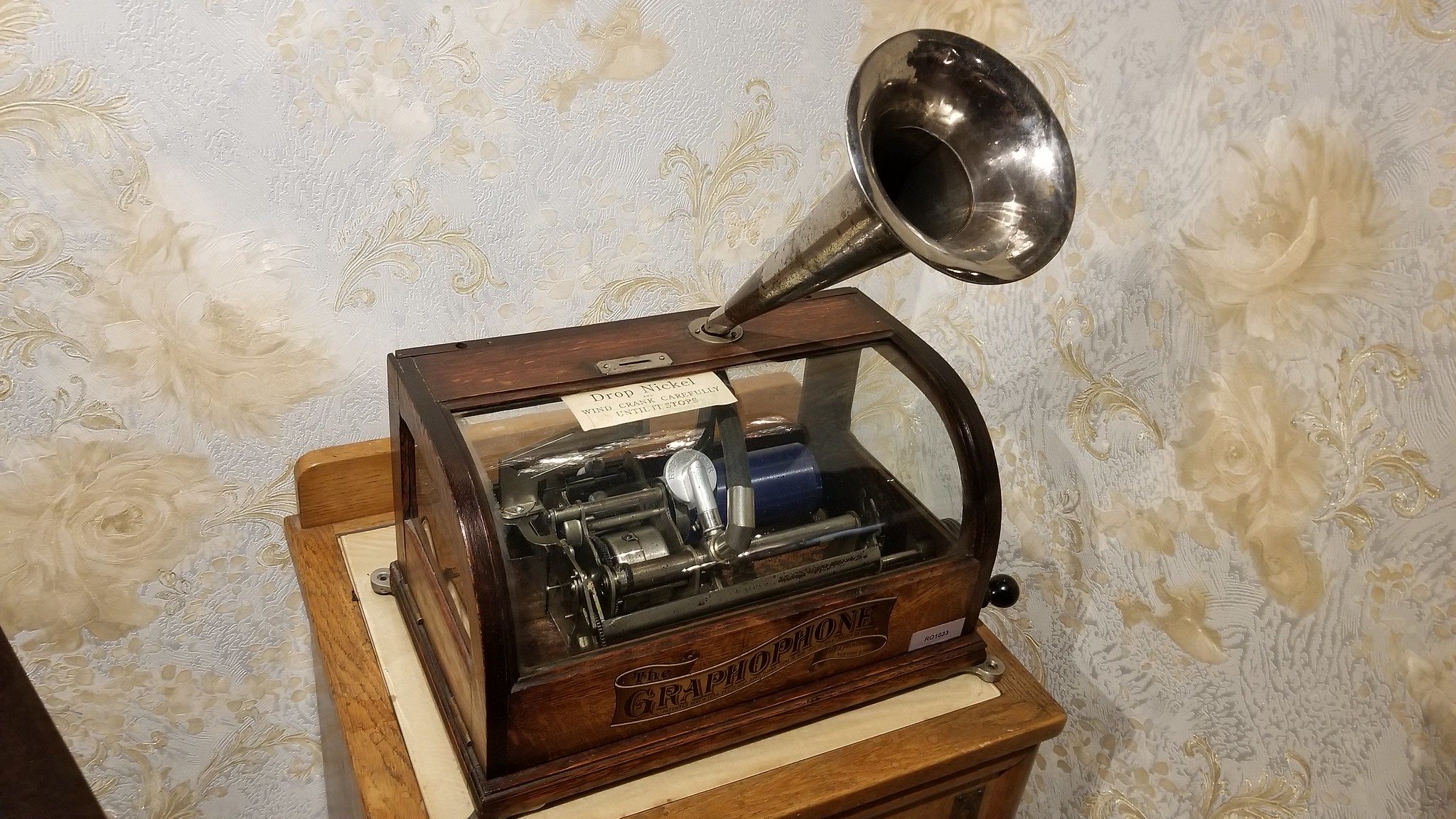The image captures a vintage graphophone, an old-fashioned musical machine encased in a wooden box with a curved glass front. A prominent brass plate reading "Graphophone" in black letters is affixed on the front. The device features a distinctive silver metal horn protruding from the top, acting as the speaker. The graphophone sits on a wooden table and has a handlebar that winds up the music. Metal components are visible inside the wooden case. The scene is photographed indoors, with the graphophone angled so the horn points towards the top of the image. The background exhibits a wall adorned in various colors, including tan, white, cream, and light blue.